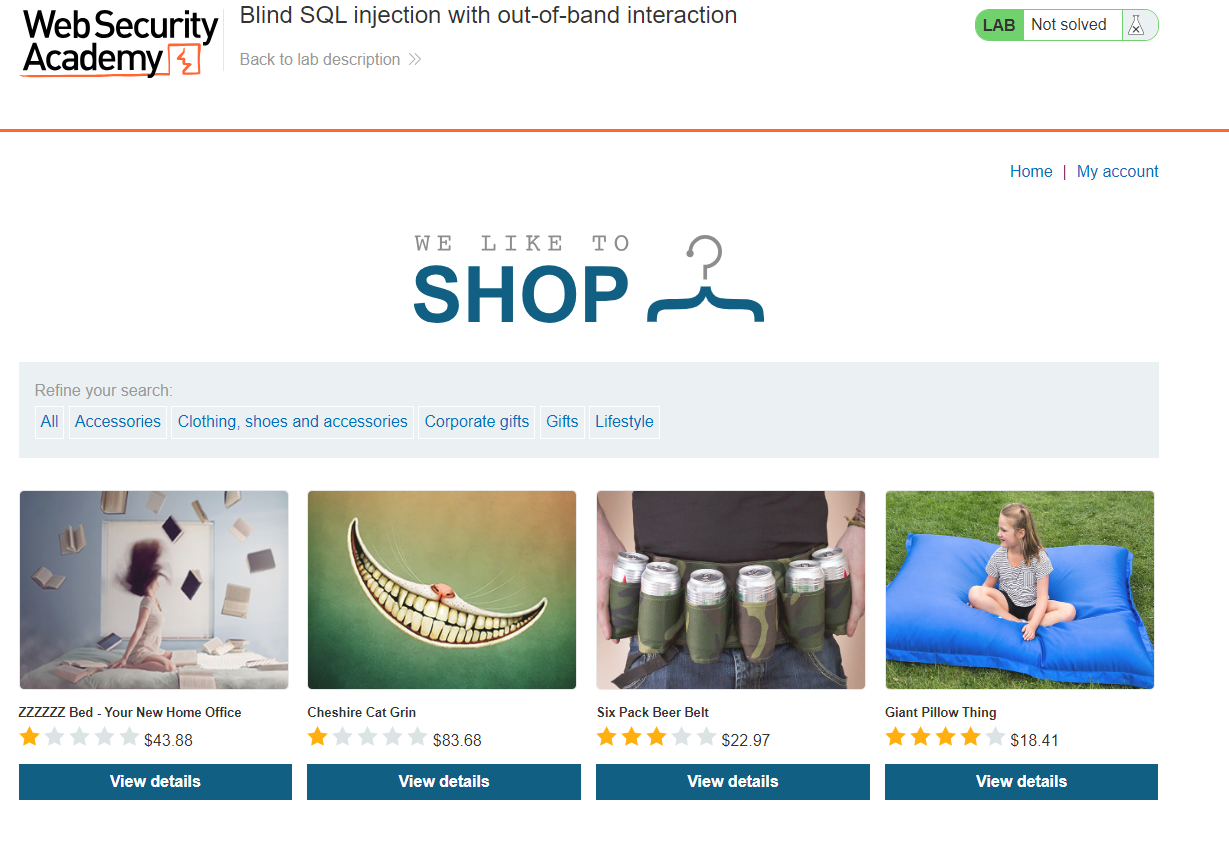The image depicts a web page from the "Web Security Academy" with a predominantly white background. At the top left corner, the website's name is prominently displayed alongside a small red icon. The page features a section labeled "Blind SQL Injection without a Band Interaction," and directly below this in faded letters, there's a link to "Back to Lab Description" marked by two right-pointing arrows.

In the top right corner, there is a segmented box with several sections. "Lab" is highlighted in green, while "Not Solved" appears in a white section next to a small gray icon resembling a test tube. Below this, a red or orange line runs across the page. On the right side of this line, the text "Home" and "My Account" appears in blue, suggesting clickable options.

Further down, a bold section reads "We Like to Shop" with "Shop" in striking blue letters, accompanied by a hanger icon. The hanger's metal hook is depicted in gray, while the bottom part matches the blue of the text. Immediately beneath this is a gray bar labeled "Refine Your Search," featuring various filters in blue text: All, Accessories, Clothing, Shoes, Corporate Gifts, Gifts, and Lifestyle.

Below these filters are four distinct sections, each linked with "View Details" in blue boxes. The items listed are "ZZZZ Bed," "Your New Home Office," "Cheshire Cat Grin," "Six-Pack Beer Belt," and "Giant Pillow Thing," each representing different product categories or options available on the website.